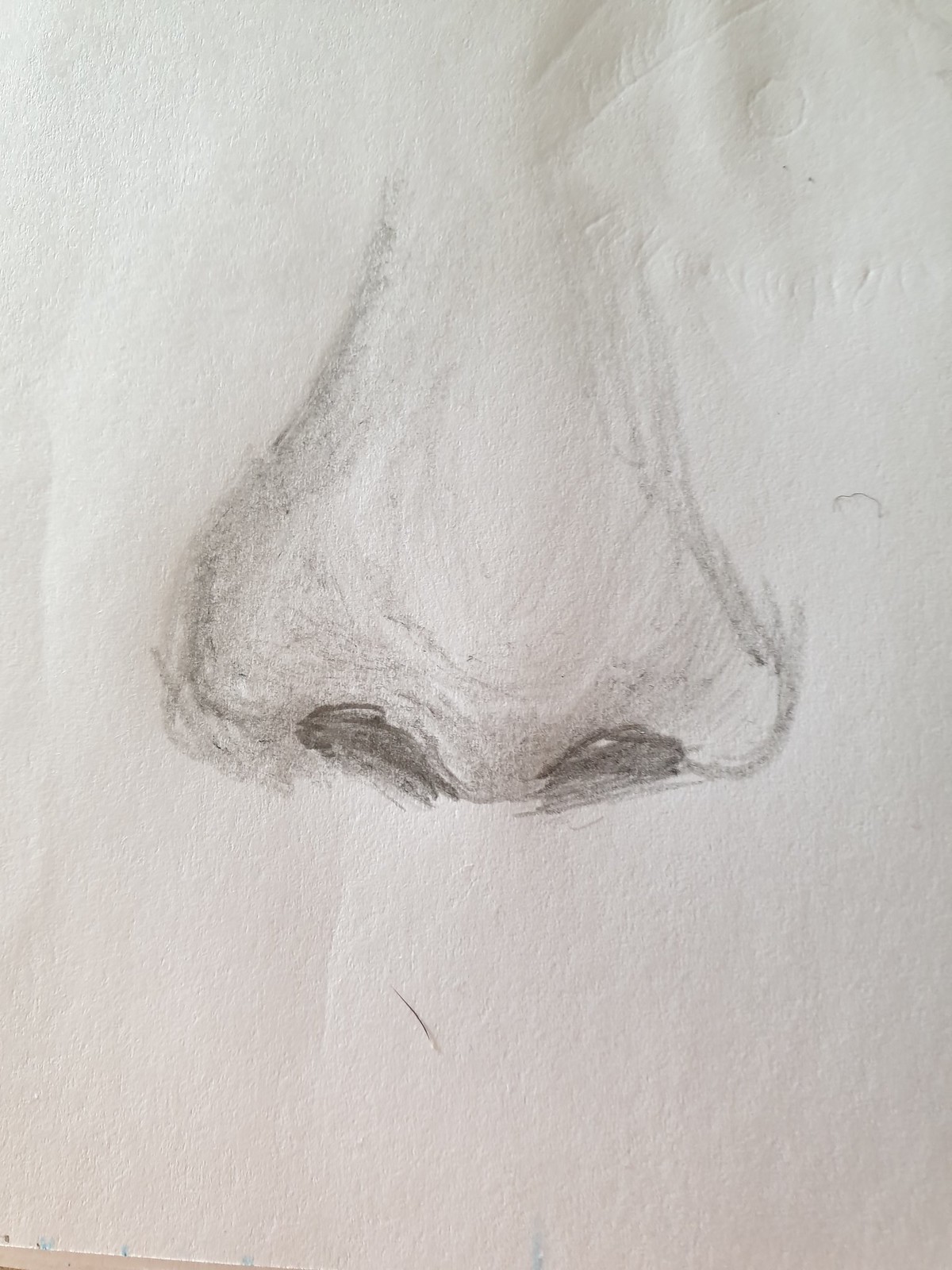The image portrays a close-up photograph of a hand-drawn sketch of a human nose, executed primarily in pencil. The sketch, oriented in portrait format, features an average-sized nose with darkly shaded nostrils and additional shading on the left side, indicating an effort to create depth and dimension. The sketch is relatively clear despite its loose, practice-oriented lines, and shows evidence of multiple outlines, possibly suggesting a study in structure or form. The rest of the sheet is blank, save for the indentation marks possibly left by drawing atop a notebook, and a single strand of real black hair resting at the bottom of the page. There are no other facial features included, and no use of color within the sketch.